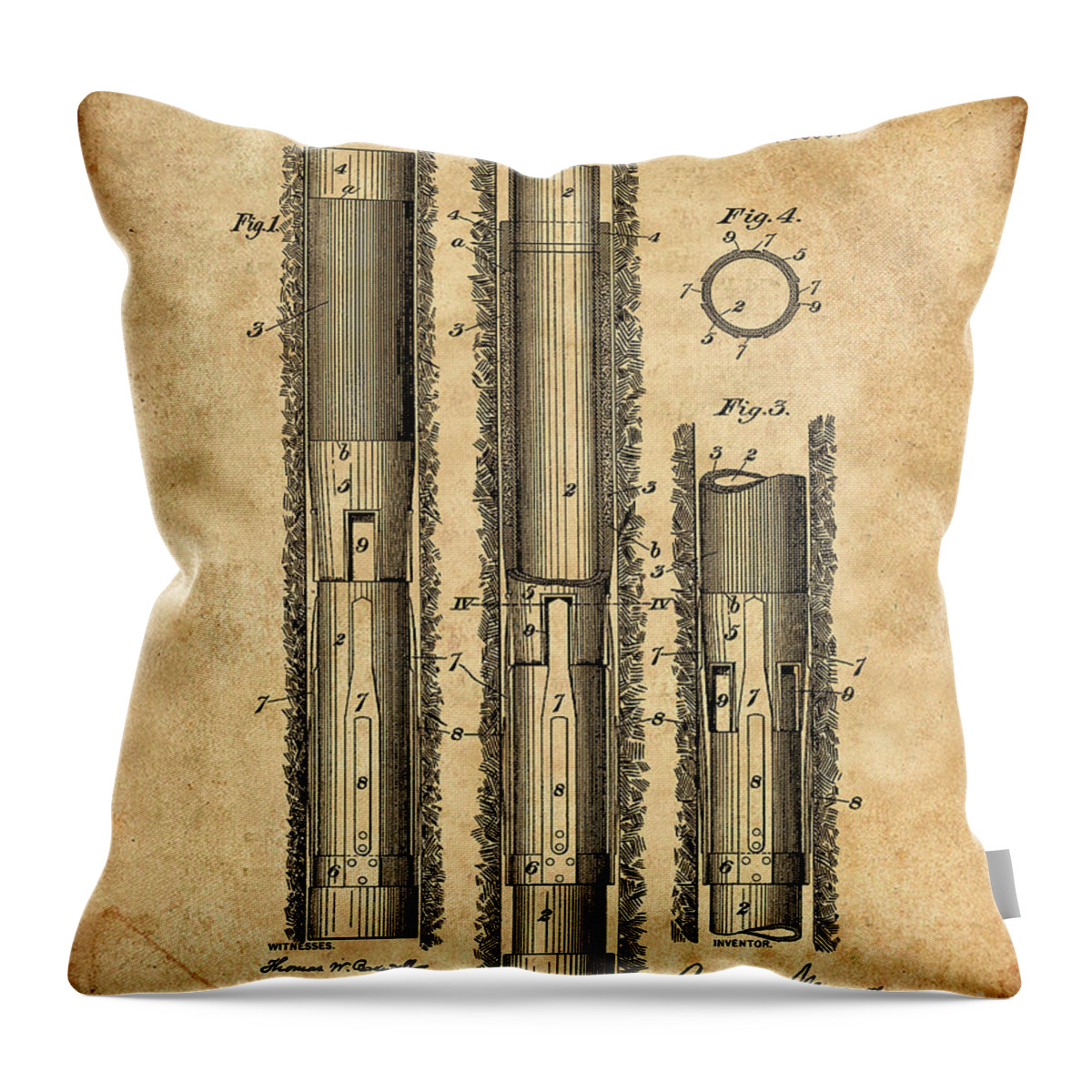The image features a decorative throw pillow standing upright against a plain white background. The pillow measures approximately four inches high and four inches wide, though its sides, top, and bottom are slightly indented, giving it an irregular square shape. It sports a light brown, blotchy coloration reminiscent of aged parchment or an old world map, with varying shades of darker and lighter brown. The surface texture suggests it might be made out of suede.

Adorning the pillow are illustrations in gray, consisting predominantly of three vertically oriented cylinders. The leftmost and center cylinders extend from the top to the bottom of the pillow, while the rightmost cylinder occupies only the upper half, with a circle labeled "Figure 4" above it. The left cylinder is labeled as "Figure 1" and is accompanied by text that reads "witnesses" beneath it, followed by an illegible cursive signature. The center cylinder, although not labeled as "Figure 2", shares a close resemblance to Figure 1. The top half of the image is occupied by "Figure 3", a horizontal half-cylinder positioned above the center cylinder.

Each of these figures has numbers such as 9, 7, 5, 2, and occasionally 3, annotated with lines pointing to various parts of the diagrams. There are also letters A and B scattered amongst the numbers. The overall impression of the imprinted illustrations is that of technical or mechanical sketches, adding a unique, almost antique aesthetic to the pillow.